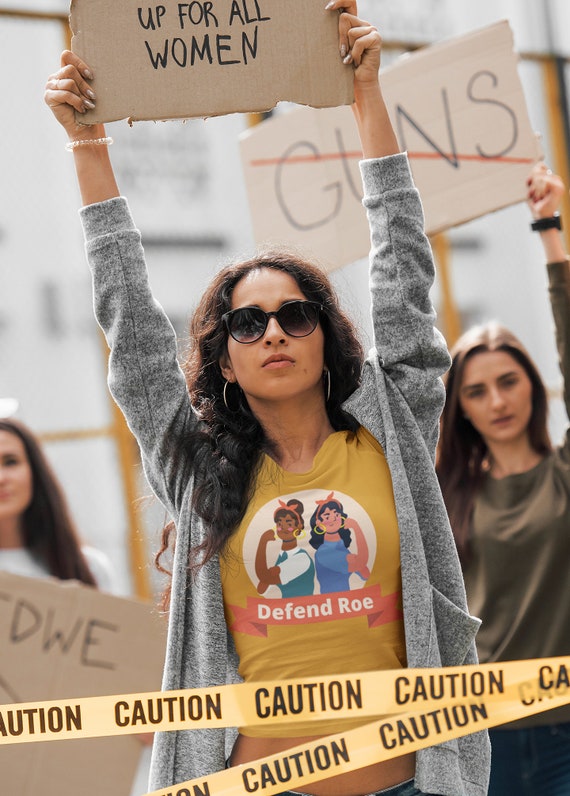The image depicts a scene at a protest featuring three women, prominently conveyed through vivid details and strong expressions. In the foreground stands a woman with long black hair, donning large silver hoop earrings and dark sunglasses, exuding a sense of determination. She wears a gray cardigan over a yellow t-shirt emblazoned with the words "Defend Roe" beneath an illustration that pays homage to Rosie the Riveter, depicting a black woman and a fair-skinned woman flexing their biceps, both adorned with red bandanas and gold earrings. Her serious demeanor adds gravity to the scene as she holds a cardboard sign aloft, reading "Up for all women," though partially obscured at the top. 

To the left of her, a partially visible woman with brown hair and light skin similarly gestures with a cardboard sign displaying the letters "DWM." On the right, slightly blurred, stands another light-skinned woman with brown hair in a dark green shirt, holding a sign that emphatically has the word "GUNS" struck through by a red line. The image is framed by yellow and black caution tape at the forefront, adding a layer of urgency and highlighting the protest's charged atmosphere.